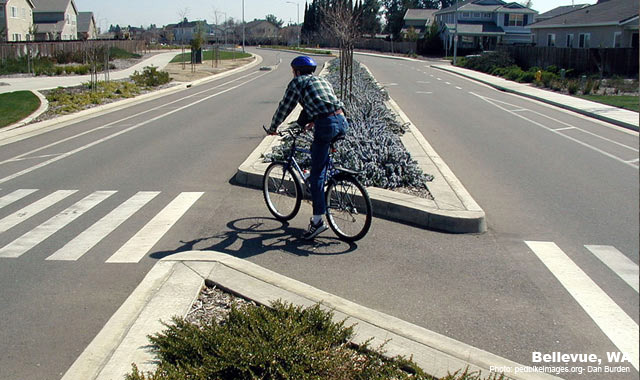This photo, taken by Dan Burden, depicts a quiet suburban scene in Bellevue, Washington. The central subject is a man, approximately 40 years old, on a bicycle positioned in the median of a two-lane road, preparing to cross the street. The cyclist is dressed in blue jeans, dark and white sneakers, a blue helmet, and a blue, white, and gray checkered flannel shirt. His left foot touches the ground while his right foot remains on the pedal, suggesting he is paused to check for traffic, although no cars are visible. 

The road features a median adorned with brown and navy blue shrubbery, dead trees, and junipers. Additional greenery, including evergreen bushes and possibly some blue flowers, can be seen in the medians, which are spaced a few feet apart. The crosswalk the cyclist is using runs through these medians, indicating a carefully designed pedestrian and cyclist-friendly area.

Surrounding the road are upper-middle-class houses, some with fences and low-growing landscaping, and newer plantings of trees. On both sides of the street are sidewalks, contributing to the residential neighborhood's accessibility and aesthetic. The background showcases a clear blue sky, adding to the peaceful ambiance of the scene. The bottom right corner of the image includes text indicating the location, Bellevue, WA, and credit for the photo to Dan Burden.